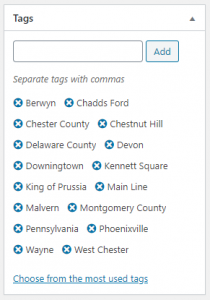The image depicts a user interface for adding tags to a phone. The outer border of the phone screen is grey, with an inner line in black, and a white background within. On the left side of the screen, there is a black font label reading "Tags," followed by a grey or black upwards pointing arrow. Directly below the arrow is a grey line, beneath which is a blank grey square. To the right of this blank square is a blue square with "Add" written in blue font against a grey background. Below these elements, in black font, are the instructions "Separate Tags with Commas."

A series of blue circles with X's beside each word represent the tags. The sequence begins with "Berwyn," followed by "Chad's Ford." On the next line below that is "Chester County," and "Chester Hill" on the same level but to the right. The next tags listed are "Delaware County" and "Devon." Below these is "Downingtown," with "Kennett Square" to its right. Further down is "King of," with "King of Prussia" directly below and to the left. Continuing, "Main Line" appears to the right of "King of Prussia." Lower on the list are "Malvern," "Montgomery County," "Pennsylvania," "Phoenixville," "Wayne," and "Westchester."

At the bottom of the image, in blue font with a blue underline, is the phrase "Choose from the most used tags."